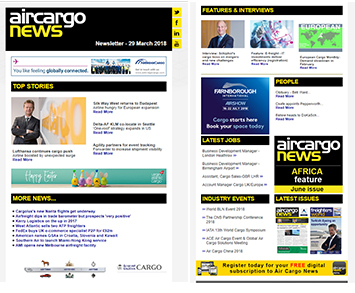The image depicts a two-page spread with varying backgrounds and a mix of text and graphics. On the left-hand page, the background is primarily black. In the upper left corner, white text reads "Air Cargo," and directly beneath it says "News." In the bottom right corner, it likely states "Newsletter," followed by the date "29 March 2018."

Four yellow icons are visible below this section. The first icon, resembling a Twitter bird, suggests social media links, followed by an 'F' likely indicating Facebook. The third icon seems to say 'LinkedIn,' while the fourth, though blurry, might represent Reddit.

As the background transitions to white, a rectangle outlined in a teal color appears. Within this area, there's a magenta figure which is unclear—it might be an airplane, an arrow, or a bird. A line of the same magenta color stretches horizontally within the rectangle, accompanied by indistinct words in teal.

Beneath this section, a black background reappears with the yellow text "Top Stories." A man in a suit with folded arms is pictured here, though the surrounding words are unreadable. There is a small green section with white text that appears to say "Happy Easter."

On the right-hand page, a yellow text box labeled "Features and Interviews" is visible. Adjacent to this are images: one of another man, some animated graphics, and a green-and-gray map.